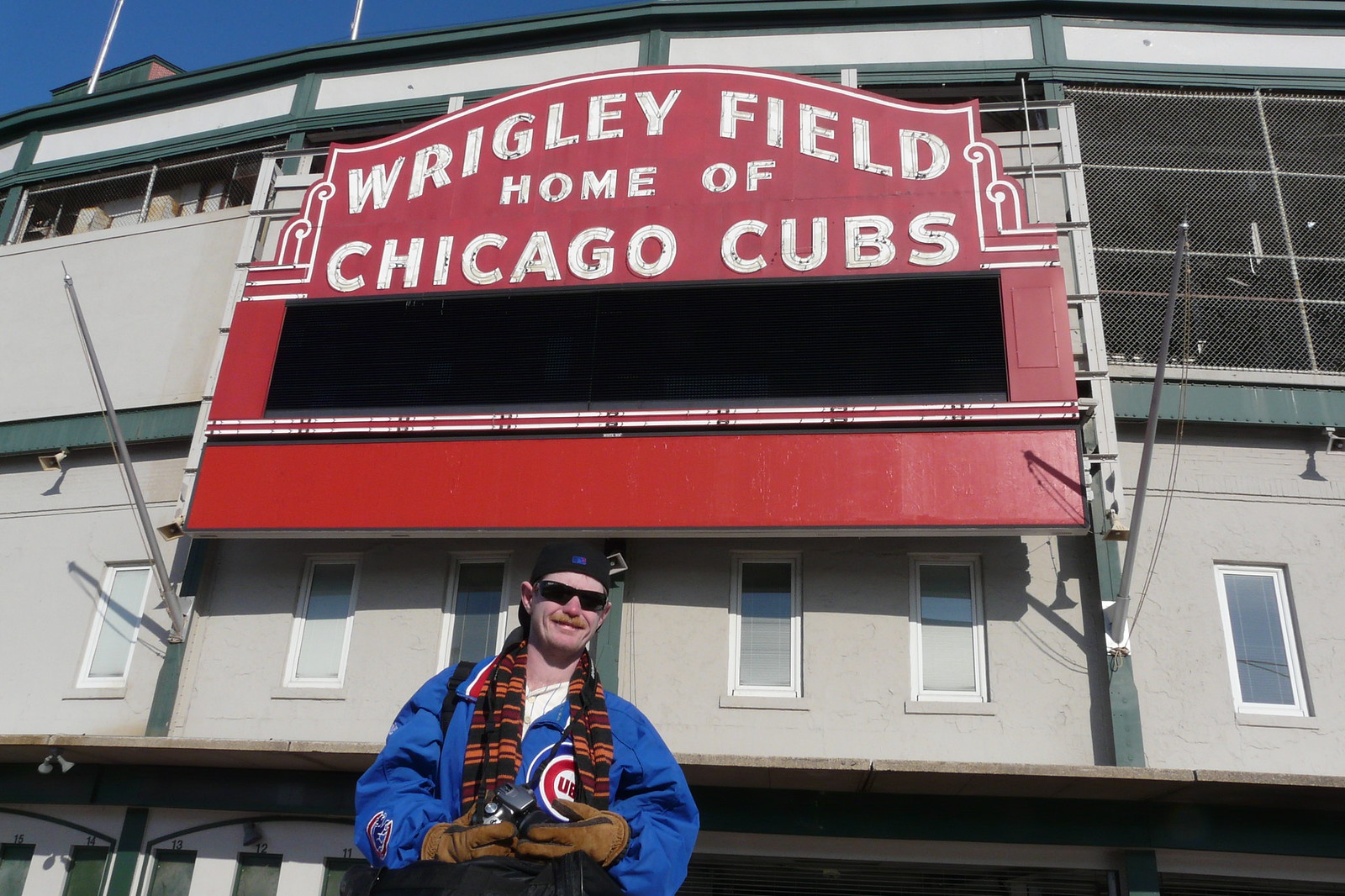The image is a color outdoor daylight photograph of a fair-skinned man posing in front of Wrigley Field, the iconic sports stadium in Chicago. He is positioned at the bottom center of the image, directly beneath a large, prominent red sign that reads "Wrigley Field, Home of Chicago Cubs" in white lettering. Below this sign is a black rectangle, likely an unlit digital display.

The man is dressed warmly, wearing a blue jacket with a circular Cubs logo on the right side of the chest, featuring blue and red circles and the word "Cubs" in the center. Partially obscuring the logo, he has a scarf around his neck adorned with black, orange, and amber-colored vertical stripes. He is also wearing thick, heavy brown gloves and a gray baseball cap turned backwards. His facial features include a light brown mustache and dark black sunglasses.

In the background, the wall of Wrigley Field is visible, displaying a light gray color with numerous white-framed windows. Green structural supports run across the building, and the upper right section of the image features a chain-link fence over a large opening. The upper left of the image shows a clear blue sky and the bases of tall flagpoles extending above the stadium's facade. Overall, the photograph captures the essence of a historical sports venue with a dedicated fan proudly standing in front.